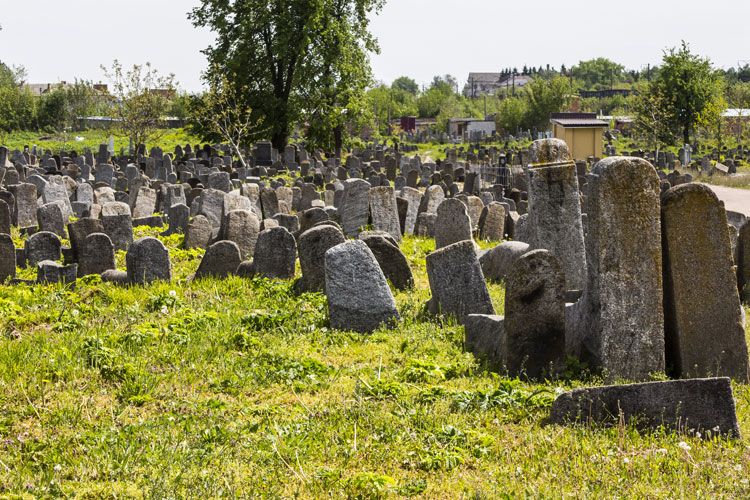The photograph captures a densely clustered cemetery on a sunny day, likely situated in a rural area. The scene is chaotic, with numerous gray concrete headstones packed closely together, many leaning or slanting as if succumbing to the passage of time. Weeds sprout abundantly among the unkempt green grass that blankets the ground. In the distance, a picturesque landscape unfolds, featuring multiple trees lining the horizon and adding a sense of serenity. To the right, a small yellow building with a brown roof stands prominently, while further beyond, houses are nestled on a hill amongst the tree lines, suggesting a quaint, possibly foreign, countryside setting.